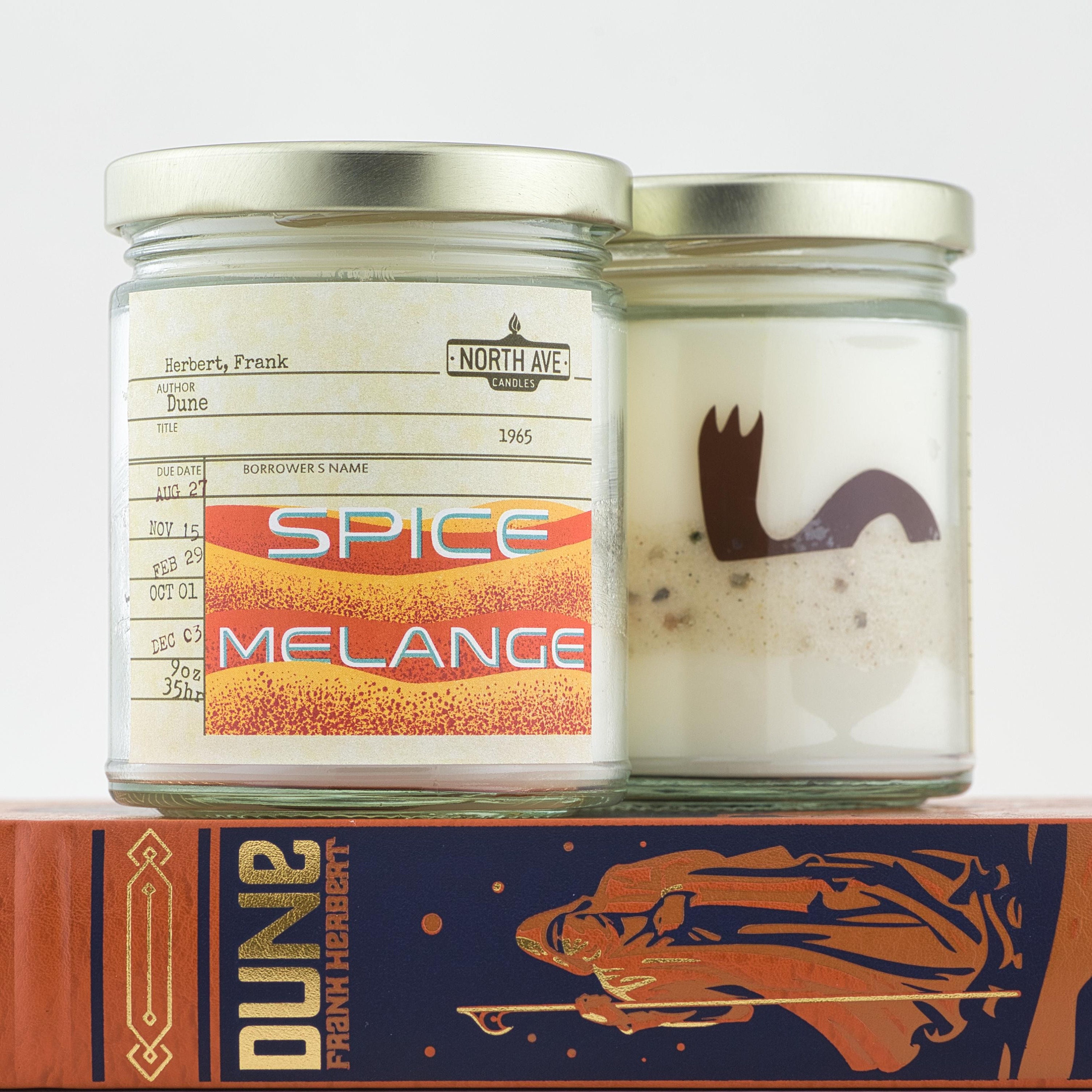The image features two glass jars and a box, all intricately themed around Frank Herbert's "Dune." The jars, both with silver metal lids, sit atop a box that is predominantly colored in shades of gold, orange, and navy blue. 

The jar on the left displays an orange and yellow desert-like design with the label "Spice Melange." Beneath this, a white sticker with black text reads "Herbert, Frank, author Dune 1965," along with "North Avenue Candles." This label is styled like a library card, complete with multiple due dates, including August 27th, November 15th, February 29th, and more, though some dates are partially obscured.

The jar on the right is filled with a white substance and features a brown squiggly line, evocative of the giant sandworms from the "Dune" universe. The background showcases a blue-purple box adorned with celestial circles resembling planets or stars. The box is titled "Dune" in gold lettering, with "Frank Herbert" written in orange beneath. The box artwork includes a robed figure with a hooded head, face obscured, carrying a large staff, further reinforcing the "Dune" theme.

Overall, the image vividly captures elements from the "Dune" series, blending literary and cinematic motifs to create a richly detailed composition.